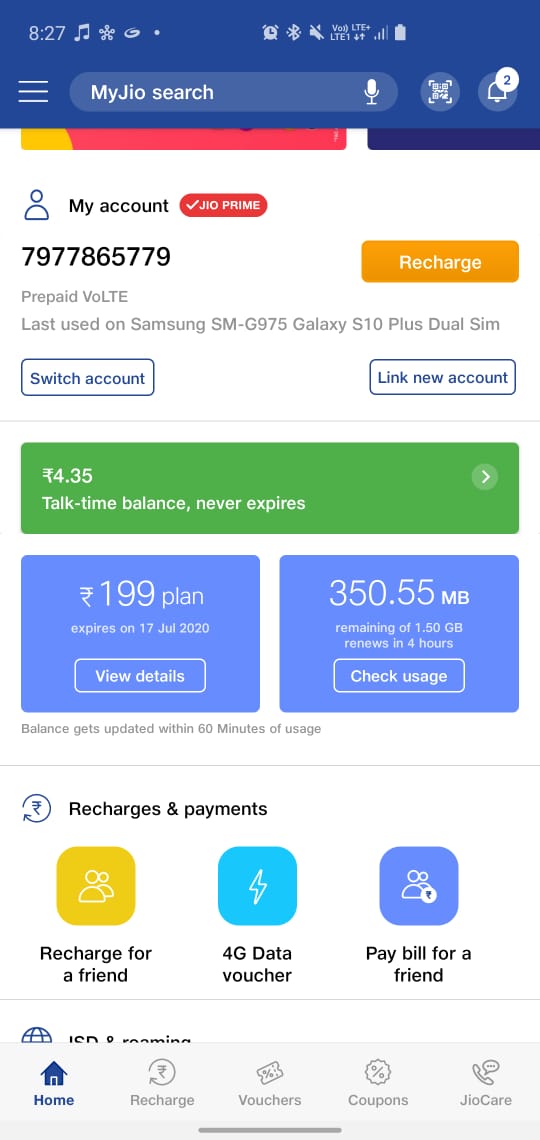This is a detailed screenshot of an account page from a mobile app. 

At the top of the screen, a dark blue header spans across, featuring three horizontal white lines stacked vertically on the left side. Directly to the right of this, there is a medium gray search bar with rounded edges, containing white text that reads "MyGeoSearch" with a capital M and J. At the far right of the search bar, there's a white microphone icon. 

The main section of the webpage is primarily white. In the upper left corner, a blue generic profile picture icon is displayed. To its right, black text reads "My Account," accompanied by a red badge to the right. The badge has a rectangular shape with curved edges and contains white text that says "GeoPrime" alongside a white checkmark. 

Beneath this, large black text displays the phone number "7977865779." Adjacent to this number, there's an orange button with rounded corners, featuring white text that says "Recharge." 

Below these elements, light gray text indicates "Prepaid VOLTE." Further down, in the same text style, it reads, "Last used on Samsung, SM-G975GalaxyS10 plus dual SIM." 

Underneath, there are two white buttons outlined in dark blue with corresponding dark blue text. The button on the left says "Switch Account," while the button on the right says "Link New Account."

Separated by a thin gray line, the lower part of the screen displays a large green pane with white text showing "4.35" followed by an unfamiliar currency symbol. Below this figure, it states, "Talk Time Balance Never Expires."